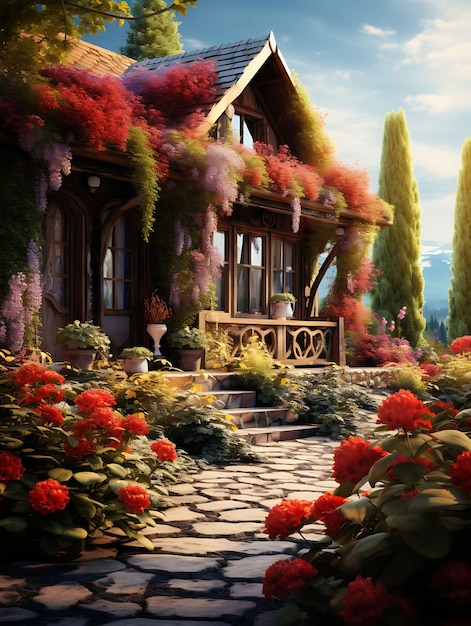The image portrays a picturesque A-frame house adorned with an abundance of windows on the front, accentuated by a small decorative wooden railing and stone steps leading up to the entrance. The roof is covered with vibrant, fluffy plants that cascade down in a mix of red, green, and pink hues. To the right of the house stand tall, pointy, and lush green trees, contributing to the serene natural setting. The sky in the background is a soft, turquoise blue adorned with white clouds, enhancing the tranquil atmosphere. A stone walkway, flanked by colorful flowers—red, yellow, and mixed green plants and stems—leads to the house, creating a warm and welcoming garden path. Additional elements include multicolored vines, such as green, red, and purple, sprawling across the house, and potted plants adorning the porch. The multitude of flowers and diverse plant life surrounding the house, combined with the vivid array of colors in the image—including red, green, blue, purple, gray, black, and yellow—offer a visually rich and inviting scene. There are no people in the image, allowing the focus to remain solely on the charming house and its lush, meticulously cared-for garden.